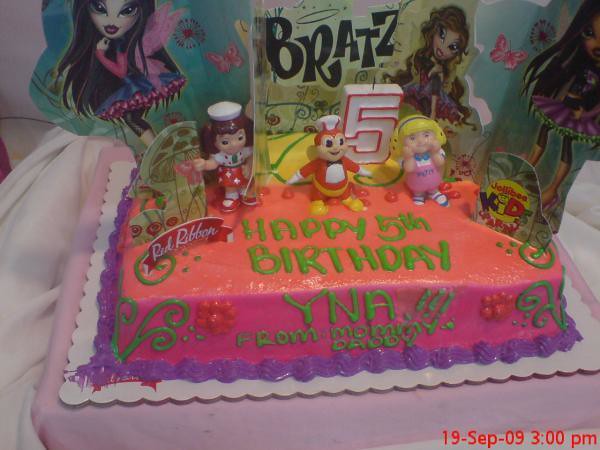This is a detailed colour photograph of a birthday cake for a five-year-old named Yna. Taken from a slightly high angle, the cake clearly displays green piping that spells out "Happy Fifth Birthday YNA" with "from Mommy and Daddy" also written in green frosting. The cake has a festive pink icing and a decorative purple border around its base. At the back of the cake, a large number five candle, white with a red outline, stands prominently. The cake features a Bratz theme, with cardboard cutouts of Bratz dolls positioned around the back and physical plastic figurines placed in front of the candle and on both sides. Additional decorations include a red ribbon banner and some green frosted stems with red flowers on the cake’s surface. The right side of the cake includes the text "Jollibee Kids," although some words are not legible. A timestamp in the bottom right corner of the image reads "19-SEP-09 3.00 PM," indicating when the photo was taken. The cake rests on a tablecloth, completing the celebratory scene.